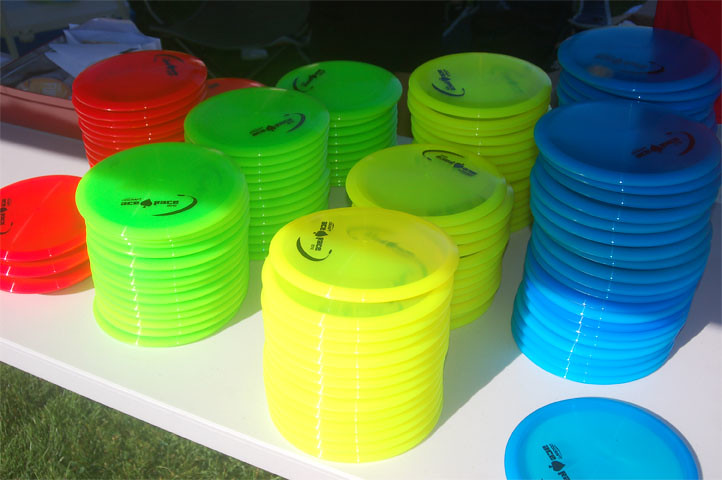This outdoor photograph captures a long white plastic table positioned on green grass, likely under an event tent on a sunny day. The lower left corner of the image shows grass, while the top part is shadowed and dark. On the table are neatly organized piles of frisbees in varying colors, each adorned with a corporate logo printed in black, though the text is unreadable from this distance. From left to right, there are three piles of red frisbees, followed by three larger piles of green frisbees, three piles of yellow frisbees, and two substantial piles of blue frisbees. Additionally, one lone blue frisbee sits at the bottom right-hand corner of the table. The arrangement suggests these frisbees are being distributed at a corporate or sporting event.